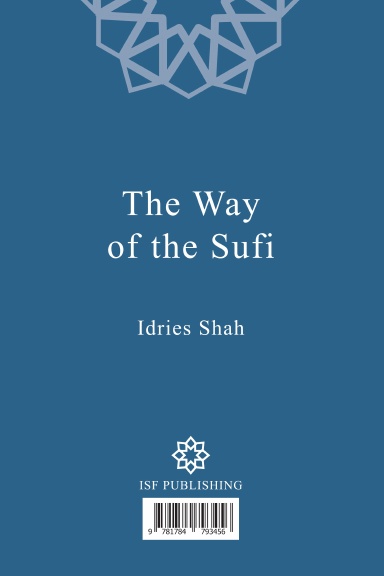The image is of the back cover of the book "The Way of the Sufi" by Idries Shah. The cover features a darker blue background with white text. At the top, there is a partial ISF Publishing logo, comprised of geometric or possibly floral shapes, rendered in gray. The book's title, "The Way of the Sufi," and the author's name, "Idries Shah," are centrally aligned in the middle of the cover in white text. Below the text, at the bottom, is another ISF Publishing logo, followed by a barcode with the number 9781784793456. The design elements on the cover, including the geometric shapes and text, provide a clean and organized layout.